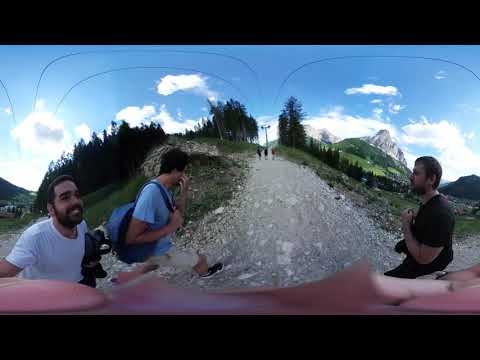The photograph captures a picturesque hiking scene on a rocky, light brown walkway that gently slopes upward, winding through a mountainous landscape. On the right side of the pathway, a man with dark brown hair and a dark shirt stands facing left, his hand raised in front of his chest, possibly holding a camera for a selfie. To the left, two men are captured: the first wears a blue shirt and a dark blue backpack, facing right but looking up the path, and behind him is a smiling man with black hair, a black beard, and a white shirt. Further along the dirt and rocky trail, three more hikers walk in the distance.

Towering green trees flank the pathway on either side, under a sky that transitions from a clear blue to scattered gray and white clouds. Among these clouds, a bright burst of sunlight shines through, particularly prominent on the left. Far up the trail, an antenna with two outward-facing wings stands at the center, a distant landmark amidst the lush greenery. The photo, likely taken with a wide-angle camera given the arcing lens lines visible in the sky, captures the natural beauty and the camaraderie of friends hiking up towards the majestic, possibly snow-capped mountain in the far background.